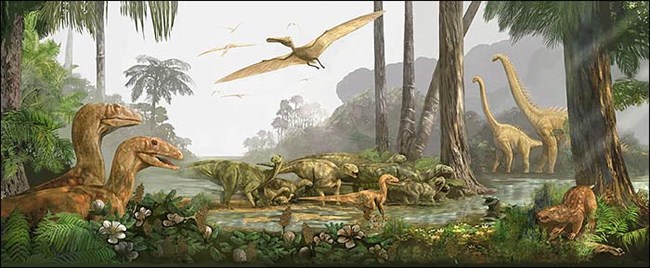The image is a detailed painting depicting a prehistoric scene teeming with diverse dinosaur species in their natural habitat. Central to the composition is a pond surrounded by lush green vegetation, including palm trees and other foliage. Several types of dinosaurs are present, showcasing a variety of behaviors and interactions. In the background, two large Brontosauruses, identifiable as a male and female, are situated on a small island, extending their long necks to feed on leafy branches. Flying overhead are several Pterodactyls, resembling large bats, gliding effortlessly through the air.

Amidst the greenery around the pond, medium-sized dinosaurs, including Velociraptors, can be seen among the dense plants and grass. On the edge of the pond, a formidable Tyrannosaurus Rex lurks, adding a sense of predatory tension to the scene. In the bottom right corner, a tan saber-toothed tiger with white stripes and a short tail crouches by a tree, observing its surroundings cautiously. Additionally, a small, brown, furry mammal is depicted on the side next to a tree, hinting at the variety of life forms present during this era.

The painting, while not vividly colorful, captures a serene yet dynamic moment in prehistoric times, emphasizing the rich biodiversity and complex interactions of ancient ecosystems.